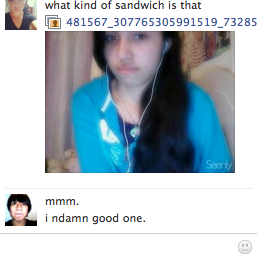This image is a screenshot from a social media platform, possibly something similar to MySpace or an older version of Facebook. The screenshot captures a conversation about a sandwich. The top half of the image features a profile picture and handle of an Indian girl with dark brown hair, wearing corded white earbuds. She has a scowling expression and above her picture, in black text, she asks, “What kind of sandwich is that?” Below her question, there is a longer string of numbers, likely representing a file name. The bottom half of the screen shows a response from another user, an Indian teenage boy with black hair, who comments, “A damn good one,” possibly in response to her query about the sandwich. In the bottom right corner of the image, there is a small smiley face watermark.